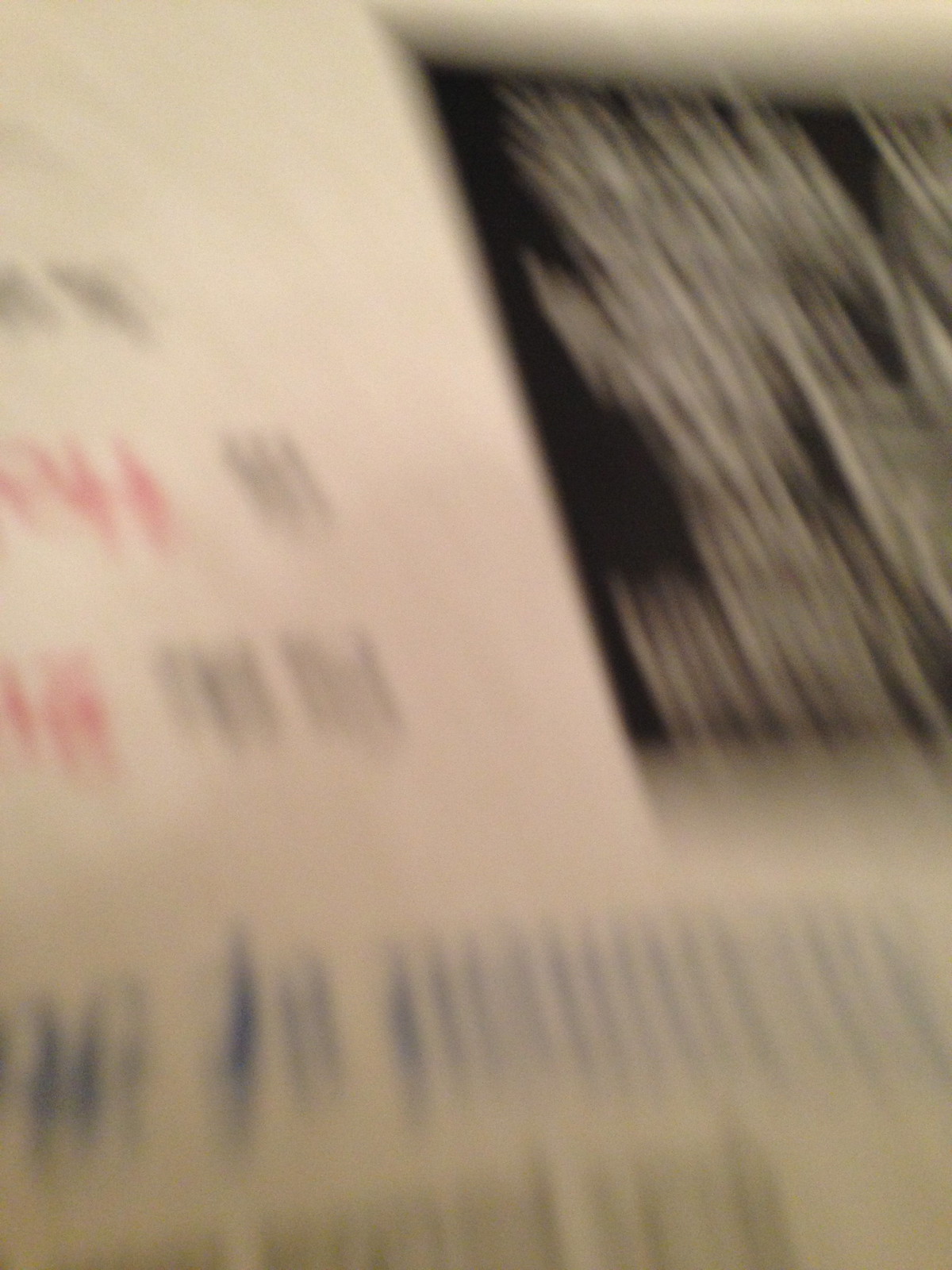An indoor color photograph, taken in low light, depicts a cluttered desktop covered with various papers. The image is blurred, with a dim ambiance that obscures much of the detail. Positioned left of center is a white sheet of paper featuring black and red print. During the lower third of the image, a light tan piece of paper, overlaying the white sheet, displays a blueprint. In the upper right, a black square piece of paper with indistinct white print appears to be streaked with blurring that runs diagonally from the upper portion to the lower right. The upper right corner of the image is dominated by a white expanse, possibly the ceiling or another piece of paper. Although some text and print are visible on these documents, they are illegible due to the significant blur. The black paper is situated to the right, and the white paper is to the left in the upper portion of the photograph.